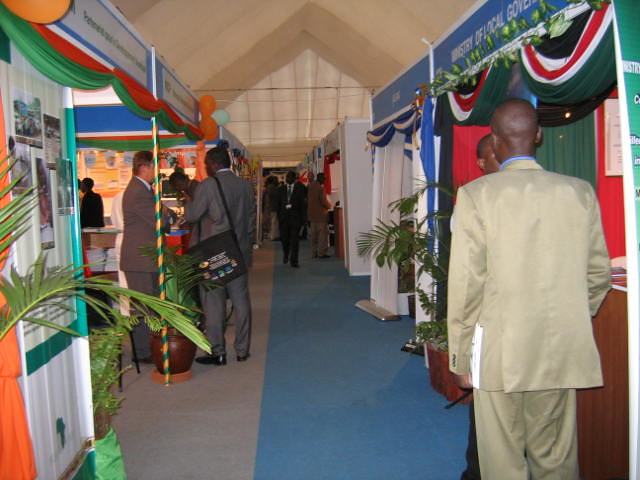This image depicts the interior of a large, peaked-roof structure, possibly a tent, with high ceilings where beams converge at the top. The floor is divided by a central seam, with gray carpet on the left and blue carpet on the right. The space is lined with square booths on either side, each booth adorned with curtains that are drawn back to allow entry. Above the booths, there are decorative banners or streamers hanging down. 

In the foreground, two men in suits are conversing; the man on the left is facing right, and the man on the right, who has a black bag slung over his shoulder, is facing away and to the left. Further down the aisle, another man in a light-colored suit faces away, talking to someone whose face is partially visible over his shoulder. 

The photograph captures a bustling scene with several people, mostly dressed in business attire, walking and engaging in conversations. In the distance, a person walks towards the viewer along the carpeted corridor. One of the booths is labeled “Ministry of Local Government,” suggesting the setting might be an official or governmental event, potentially in Africa, as inferred from the details provided.